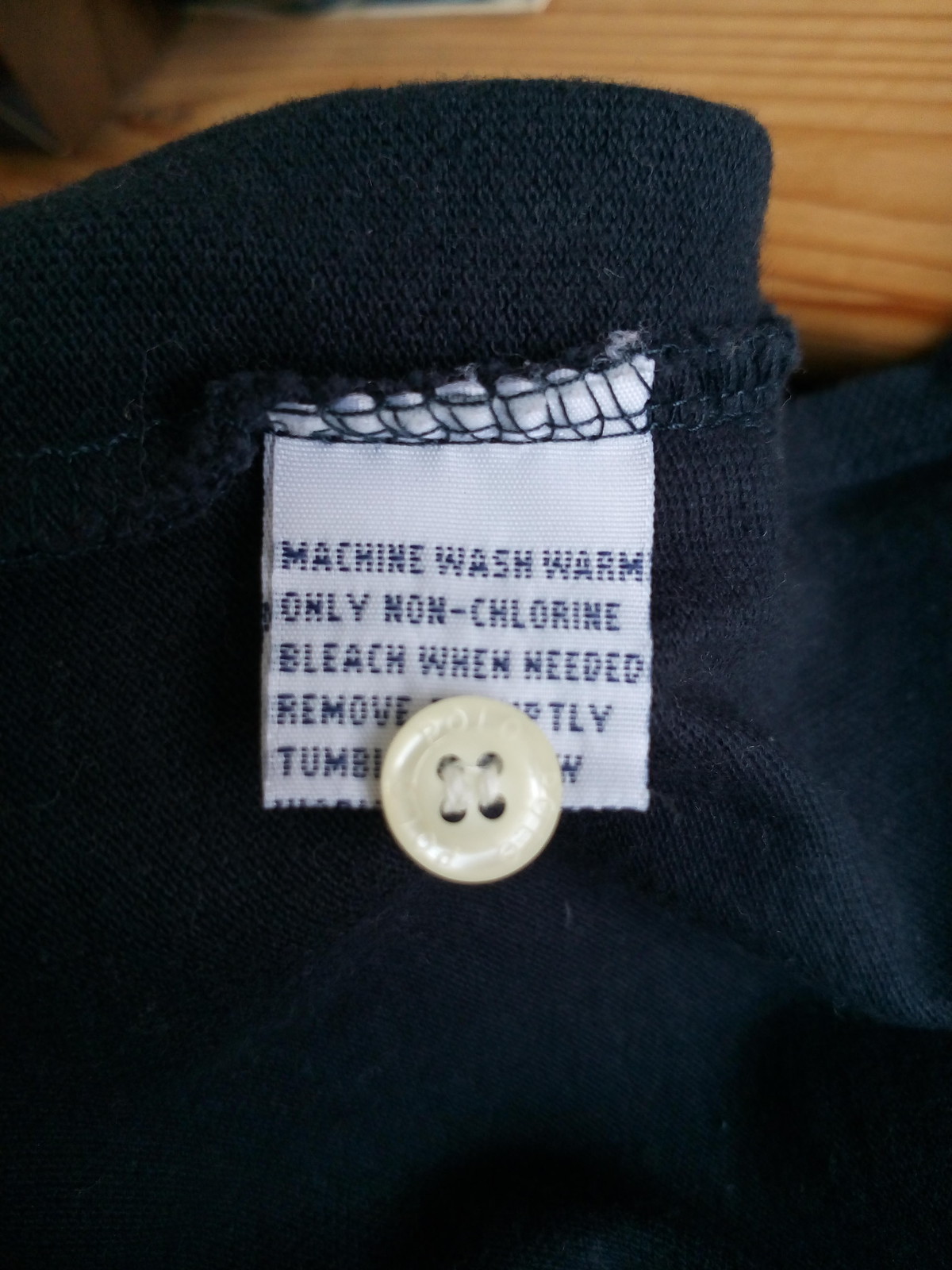This photograph features the inner tag of a knitted top, meticulously capturing the details of the care instructions label. The garment itself is a dark blue knit with a button-up design, boasting white buttons that contrast elegantly with the deep blue fabric. The focal point of the image is the white label sewn inside the top, which includes stitched text detailing how to clean the item. A spare white button is securely attached to the label, partially obscuring some of the text. The visible portion of the blue thread stitching reads: "Machine wash warm only, non-chlorine bleach when needed." The remainder of the instructions, likely about tumble drying, is partially covered by the button, making it difficult to decipher fully. The precise stitching and thoughtful addition of the spare button reflect the garment's attention to detail and quality craftsmanship.